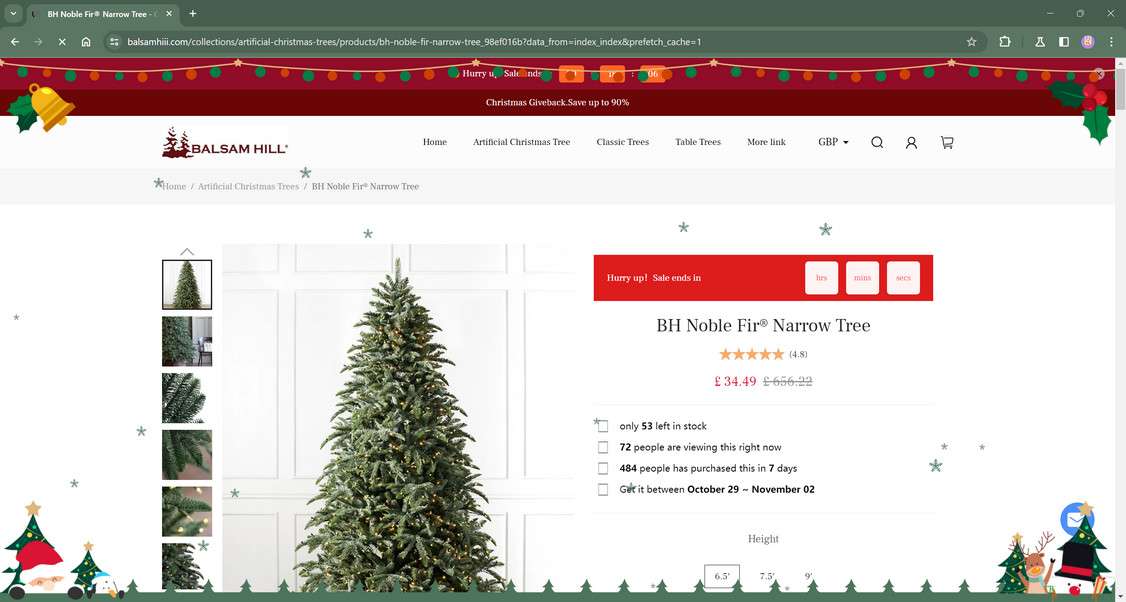This horizontal screenshot captures a desktop view of the Balsam Hill website, displayed within the Google Chrome browser, adorned with holiday-themed decorations. The URL bar at the top is colored in a festive pine green, while the navigation bar below it is a rich burgundy, embellished with a strand of lights, accentuating the holiday spirit. The specific webpage from the screenshot features the "BH Noble Fir Narrow Tree" product and displays prices in British pounds, indicating it is the UK version of the site. Additionally, festive icons are present at the bottom of the screen: a Santa icon on the lower left and a snowman head on the lower right, further enhancing the Christmas ambiance.